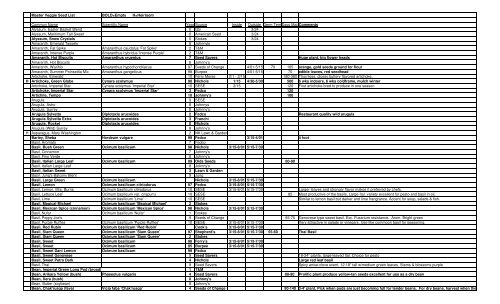This image depicts a printed spreadsheet, possibly 11 by 17 in size, containing approximately 9 or 10 columns and around 30 to 40 rows, all filled with lines of text that are too small to read. The spreadsheet features distinctively dark horizontal lines across the page. 

In the first and fourth columns, every row is completely filled, suggesting that these might contain serial numbers or other small entries. The first column is notably narrow, likely containing just numbers, while the second and third columns are wider, potentially designed for more substantial text such as first and last names. The remaining columns exhibit varying levels of detail. Some contain what appear to be words or long numbers, though the specifics are indistinct. The last column, which is notably sparse and bright, seems to hold comments or notes. Column headers are bold but unreadable, and the second and third columns also bear some labels. The spreadsheet's purpose could range from tracking login or shipping entries to listing arrival dates or cities.